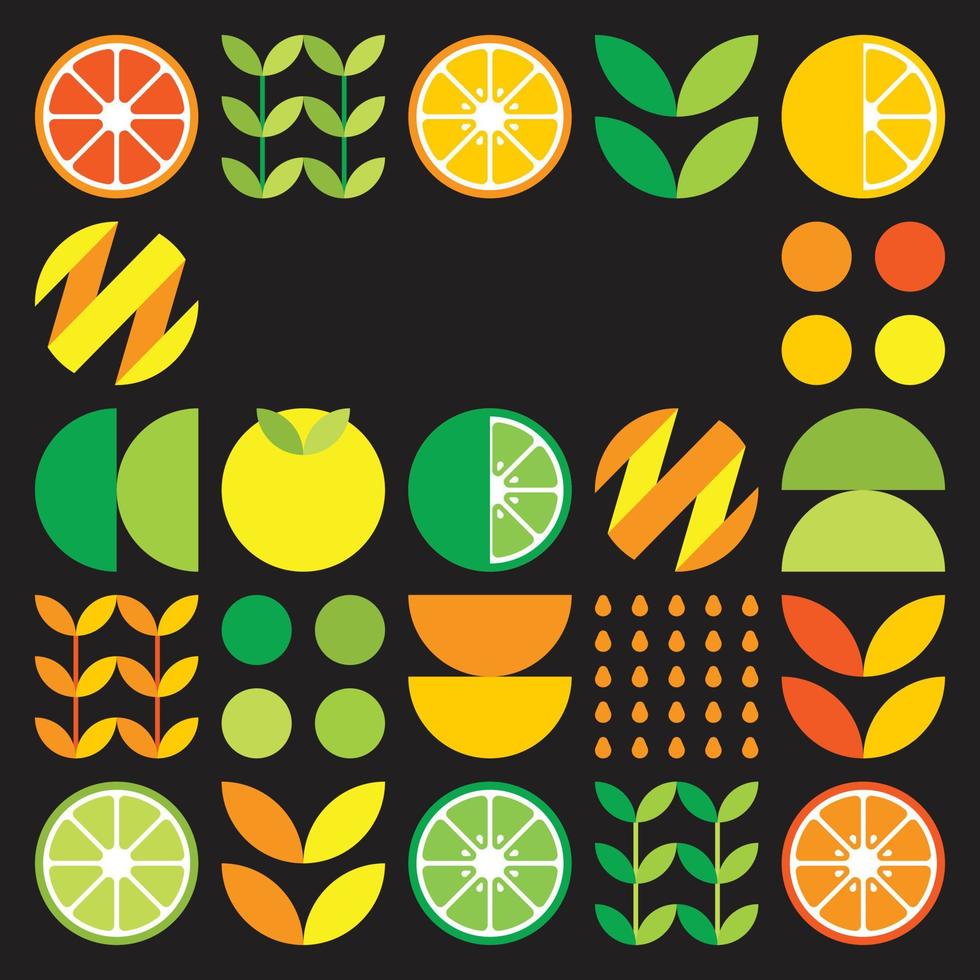The image is a vibrant, square art piece with a black background, showcasing an artistic representation of various fruits. The composition includes limes, oranges, grapefruits, and lemons depicted in multiple forms—whole, half-cut, quarter-cut, and peels. The top row features a cut-open grapefruit, some pea pods, a cut-open lemon, leaves, and partly cut oranges. In the middle rows, there are orange peels and several colored dots in shades of orange, red, yellow, and green. The bottom section continues this pattern with fruits like unpeeled lemons and additional colorful circles. The artwork also includes unique painted designs and clusters of colored dots, arranged in organized rows and columns, contributing to the overall colorful and dynamic presentation of the fruits.